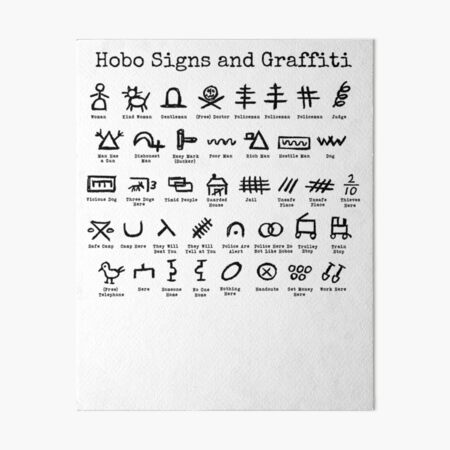This informational sheet features "Hobo Signs and Graffiti" prominently labeled in large black letters at the top against a white background. The sheet is organized into approximately five horizontal rows, each containing six or seven simplistic black-inked symbols, which hobos used during the Great Depression to communicate important information to fellow travelers about the conditions and resources available ahead. The symbols include a variety of easily recognizable drawings, such as a stick figure on a hill, a cat, a bird, a skull and bones, two shovels side by side, and a fraction (2/10), among others. Each symbol is accompanied by small black text that explains its meaning, although the writing is too small to be easily read. The bottom quarter of the paper is notably blank, emphasizing the structured layout of the signs above.